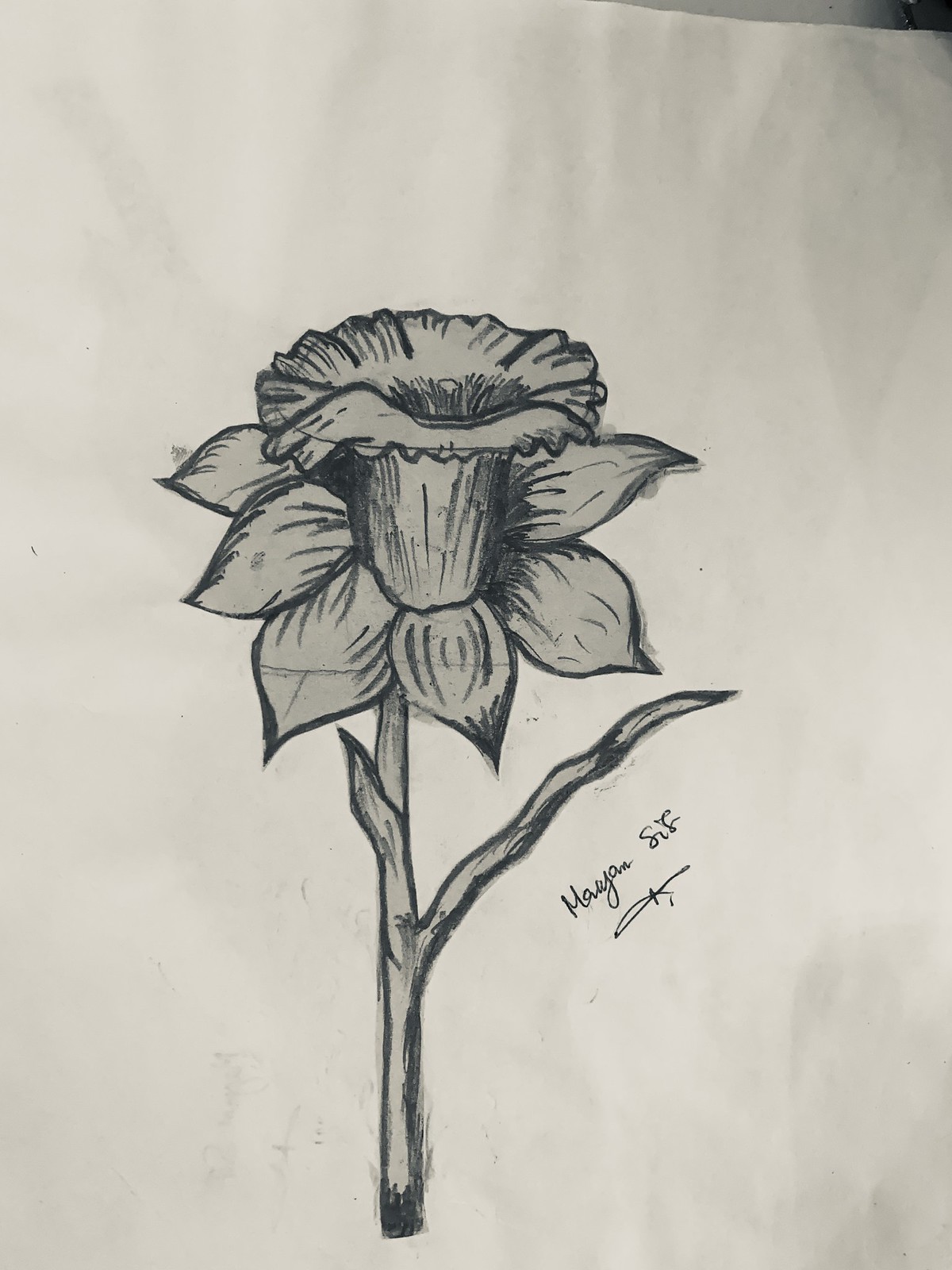This is a detailed grayscale illustration created on a piece of paper, utilizing charcoal for the primary lines and possibly watercolor or pastel for the shading. The drawing showcases a flower, likely a buttercup or another early spring bulb flower, with a distinct stem, a prominent central cup, and several auxiliary petals around it. The charcoal markings are deep black, while the lighter gray fills may be attributable to another medium like pastel or chalk. The artwork is signed, though the signature is somewhat ambiguous, potentially reading as either "Marianne" or "Megan."